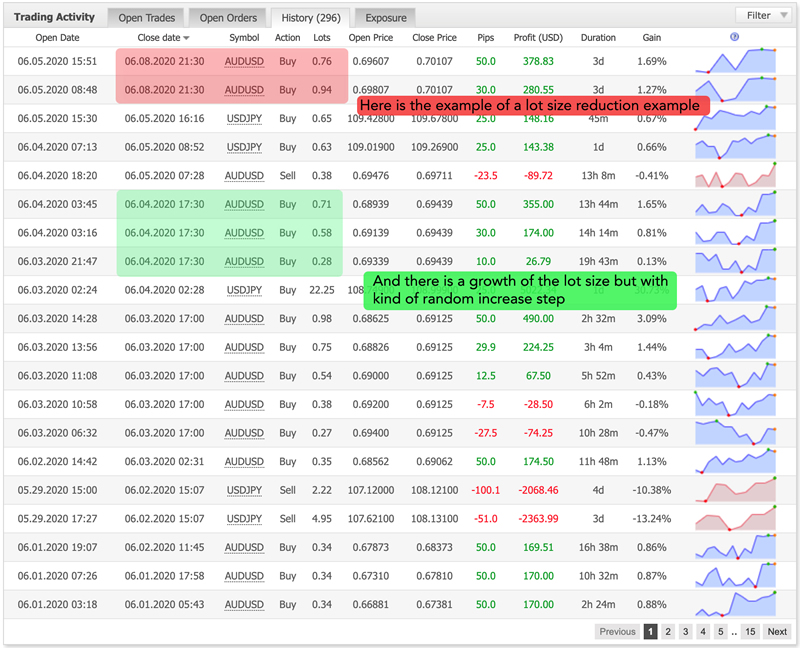This is a detailed screenshot of a trading activity page from a stock market application. At the top, the header reads "Trading Activity," and below it are several menu options enclosed in rectangles: "Open Trades," "Open Orders," "History," each with respective numbers like 298 and 296, followed by "Exposure," and on the far right, a "Filter" option accompanied by a small arrow. 

Directly underneath the "Trading Activity" header, there is a table with columns labeled "Open Date" and "Close Date," showing various dates and times such as 06/05/2020 at 15:51. The "Symbol" column lists stock market symbols like AUD/USD. The "Action" column specifies the type of action, such as "Buy," and "Lots" column indicates quantities like 0.76. 

Certain rows within the table are highlighted: two rows are highlighted in pink, while three rows below them are highlighted in green, each providing detailed trade information similar to the closed date, symbol, action, and lot size. 

Towards the center-right of the image is a prominent red line with bold black text stating, "Here is the example of a lot size reduction example," and about five rows further down appears a significant green bar with black text saying, "And there is a growth of the lot size, but with kind of random increase step."

On the right side of the screenshot, there are several graphs in blue and pink, displaying fluctuating lines that likely represent the price movements or trading volumes over time.